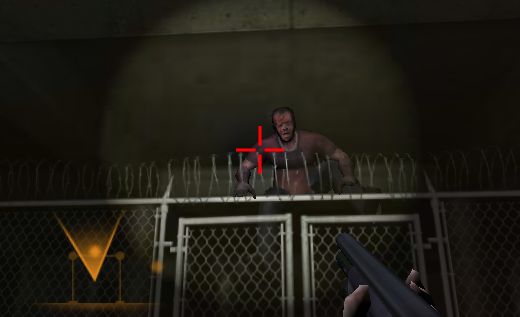This screenshot showcases a scene from a video game, depicting a first-person viewpoint. In the center, there is a red crosshair aimed through a circular focus area, with everything outside the circle appearing darker, lending a flashlight effect to the image. A character's hand, gripping a grey-black gun barrel, occupies the bottom right corner. The game environment features a silver chain-link fence with barbed wire on top, and two gates directly in front. Behind the fence is a brown-skinned character wearing a brown t-shirt, possibly appearing semi-zombie-like. In the bottom left corner, there is a graphical interface element represented by a yellow-orange arrow or circle with a grey-brown outline. The background consists of a dark green wall with a cement ceiling above it, underlining the dark and tense atmosphere of the scene.